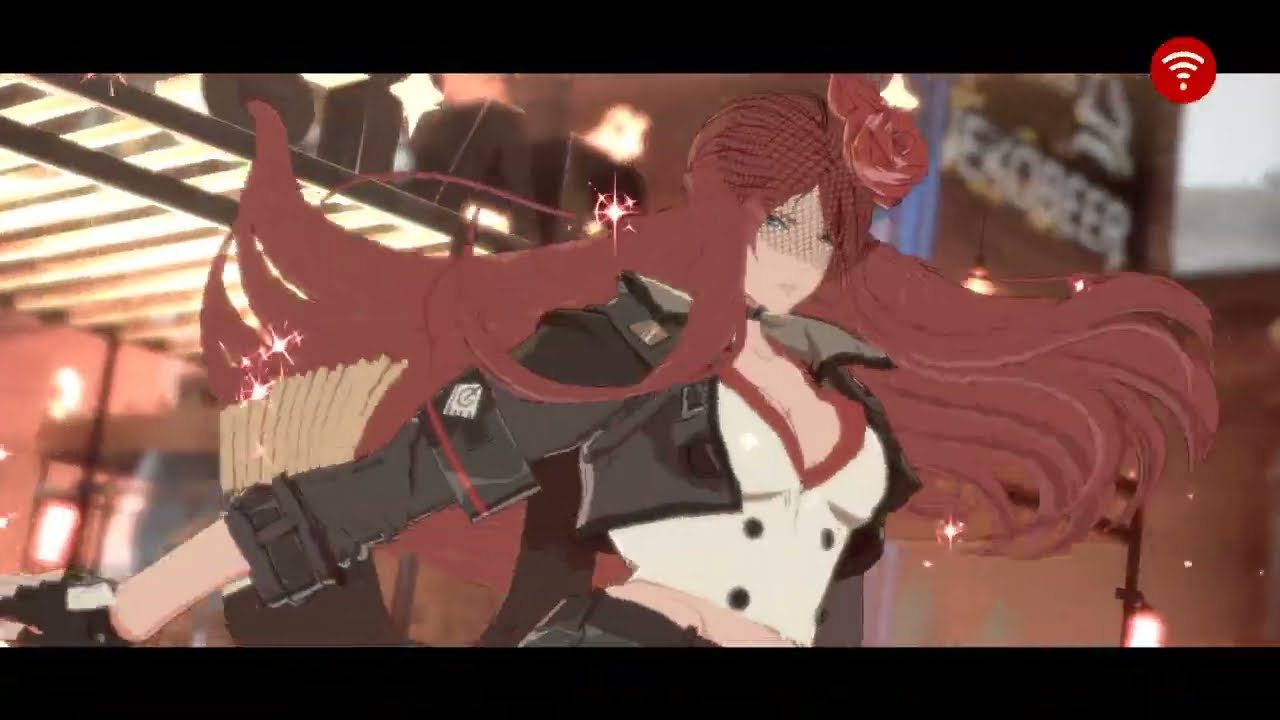The image is a horizontally rectangular, computer-generated scene, bordered by black at the top and bottom. In the top right corner, a red circle partially extends into the main area, featuring a white internet symbol. Dominating the center of the image is a striking female anime character. Sporting flowing, bright red hair that billows behind her, she is dressed in a tight-fitting white shirt with a deep V-neck and a cropped, black leather jacket with a red collar. Her right hand, adorned with a glove, extends out to the bottom left of the picture. The vantage point is from about waist height, angled slightly upward towards her face. She wears a mesh screen hat with flowers attached, adding an extra element of intrigue. 

In the backdrop, there's a cluttered industrial setting with open slats, potential staircases or walkways, and various stored boxes. Behind her to the left, an awning sign displays partially visible letters, suggesting a mix of 'A' and possibly 'R.' On the right side, amid the industrial scenery, white text on a building hints at the word "BEER." A small light fixture hangs from a pole in the bottom right corner, illuminating the scene with a convention-like atmosphere.